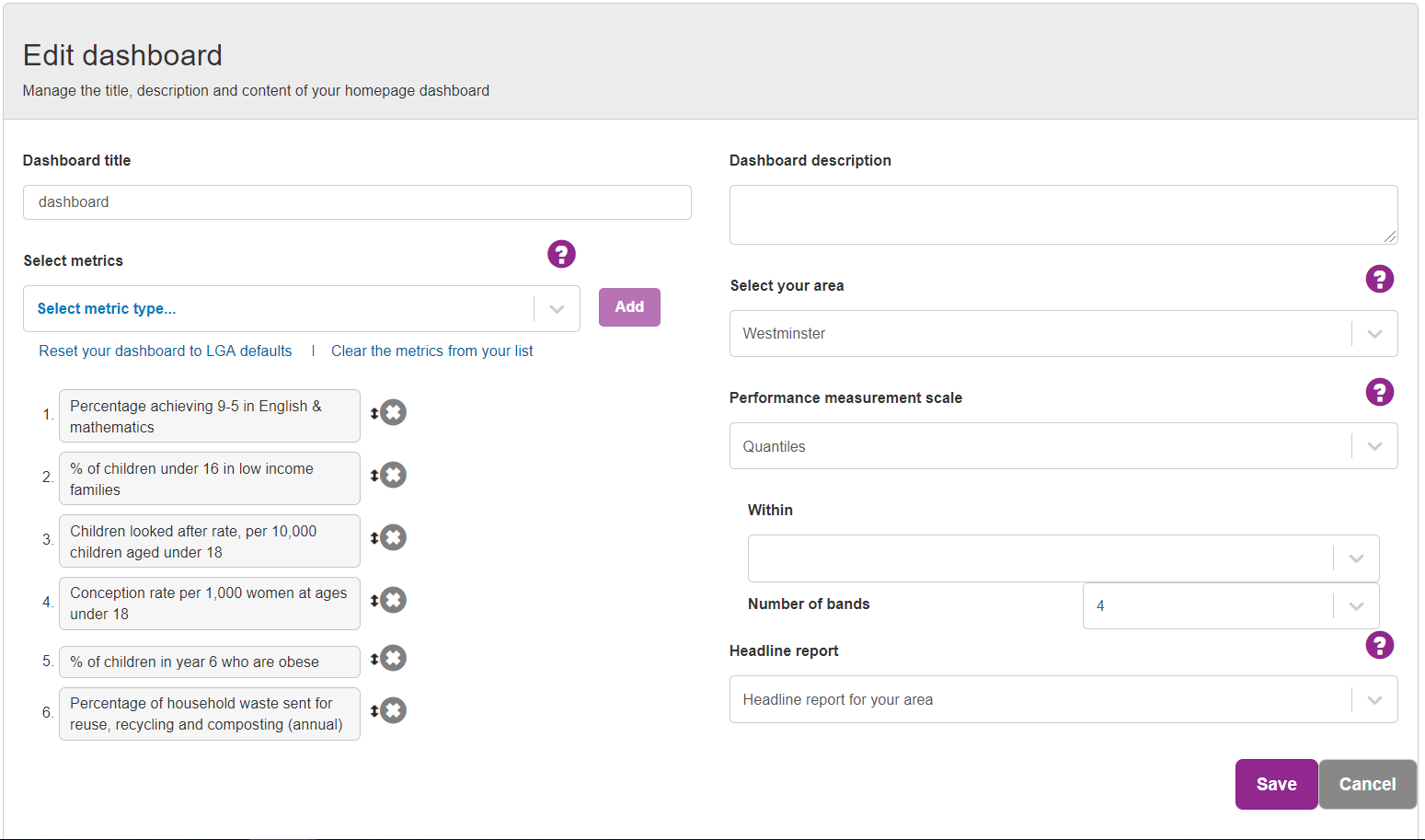This image is a detailed screenshot of a computer interface featuring a white background with black text, primarily focused on an editable dashboard setup. 

At the top, a gray navigation bar contains the text "Edit Dashboard." This section includes options to manage the title, description, and content of your homepage dashboard. 

Below this, the main white area is segmented into various input fields and options. The first section prompts the user to enter a "Dashboard Title" followed by an input box. Next, there is an option to "Select Metrics," leading to another subsection titled "Select Metric Types" where users can input their choices.

In blue text, there is an option labeled "Reset your Dashboard to LGA Defaults," followed by a line of text instructing users to "Clear the metrics from your list."

The interface is further divided into numbered metric boxes, each detailing different statistics:
1. Percentage Achieving 9-5 in English and Mathematics
2. Percentage of Children under 16 in Low Income Families
3. Children Looked After Rate per 10,000 children aged under 18
4. Conception Rate per 1,000 women aged under 18
5. [Two additional metrics follow in similar format, not entirely described in the original caption]

On the right side of the screen, there is a "Dashboard Description" field with an accompanying input box. Below this is an option to "Select your area," with "Westminster" pre-selected in a changeable field.

At the bottom right corner, there are two buttons: a purple "Save" button and a gray "Cancel" button.

This interface is designed for comprehensive customization and monitoring of various educational and social metrics, allowing the user to tailor their dashboard to specific needs and objectives.